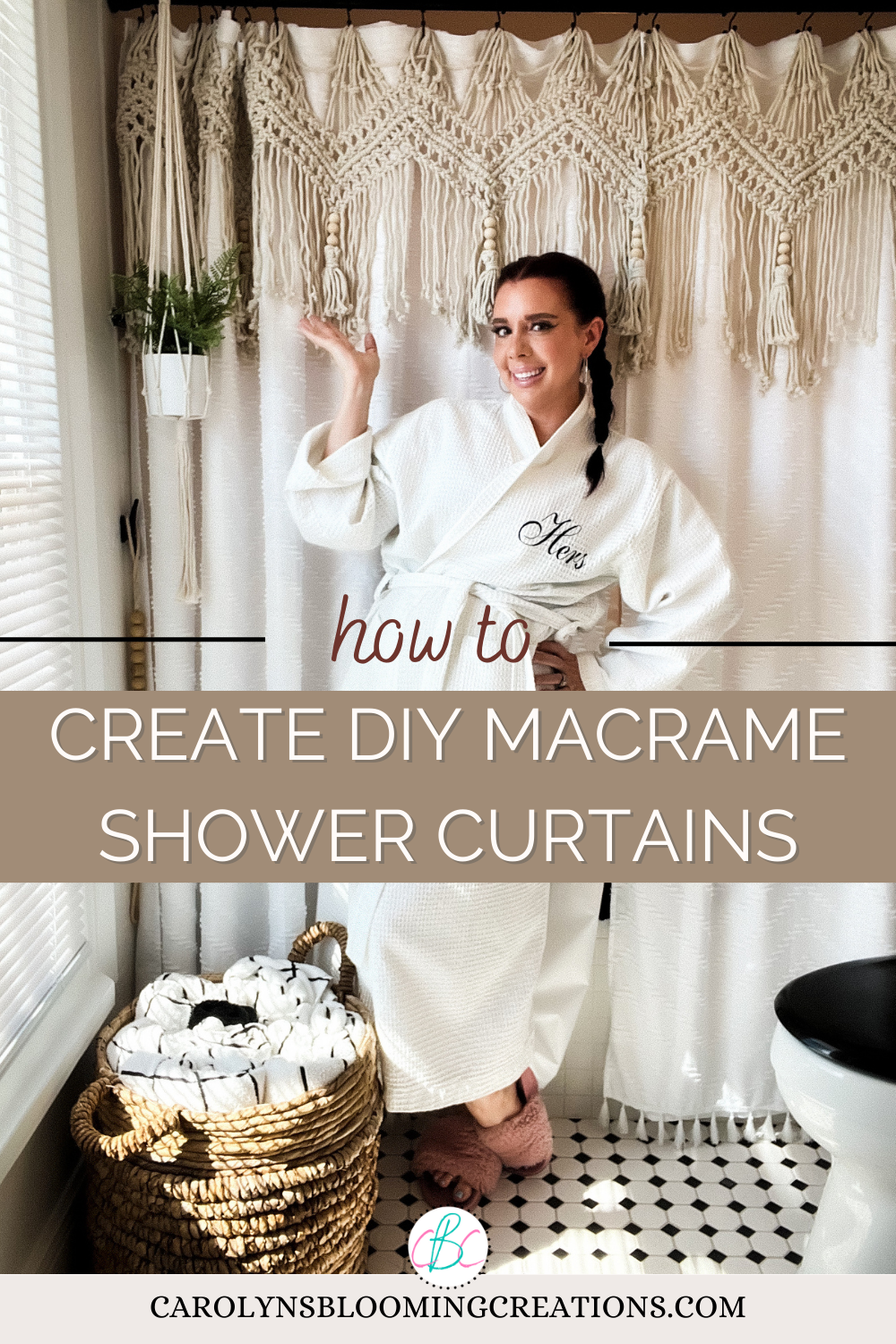The image is an advertisement in portrait layout, promoting DIY macrame shower curtains. The centerpiece of the image features a Caucasian woman standing confidently in a bathroom, with her left hand on her hip and right hand raised. She is dressed in a white bathrobe with the word "HERS" emblazoned on the chest area, and she's wearing pink slippers. Her hair is styled in braids pulled back into a ponytail.

The bathroom around her is designed with a black and white tiled floor, a white toilet with a black seat cover on the lower right, and a wicker basket filled with towels placed on the lower left. The shower curtain behind her is cream-colored with beige macrame tassels adorning the top and bottom, giving it a decorative, handmade look. Additionally, a green plant in a white pot hangs from the ceiling in the upper left-hand corner of the image.

Text overlays prominently on the image, with brown text stating "How to" positioned over her stomach and continuing with "Create DIY Macrame Shower Curtains" in white text against a brown background in the center. At the bottom, the advertisement is credited to "Carolyn's Blooming Creations dot-com" accompanied by a pink, green, and white logo. The details and composition suggest a setting that almost resembles a hotel bathroom, aimed at showcasing both the elegance and personalization of homemade macrame shower curtains.